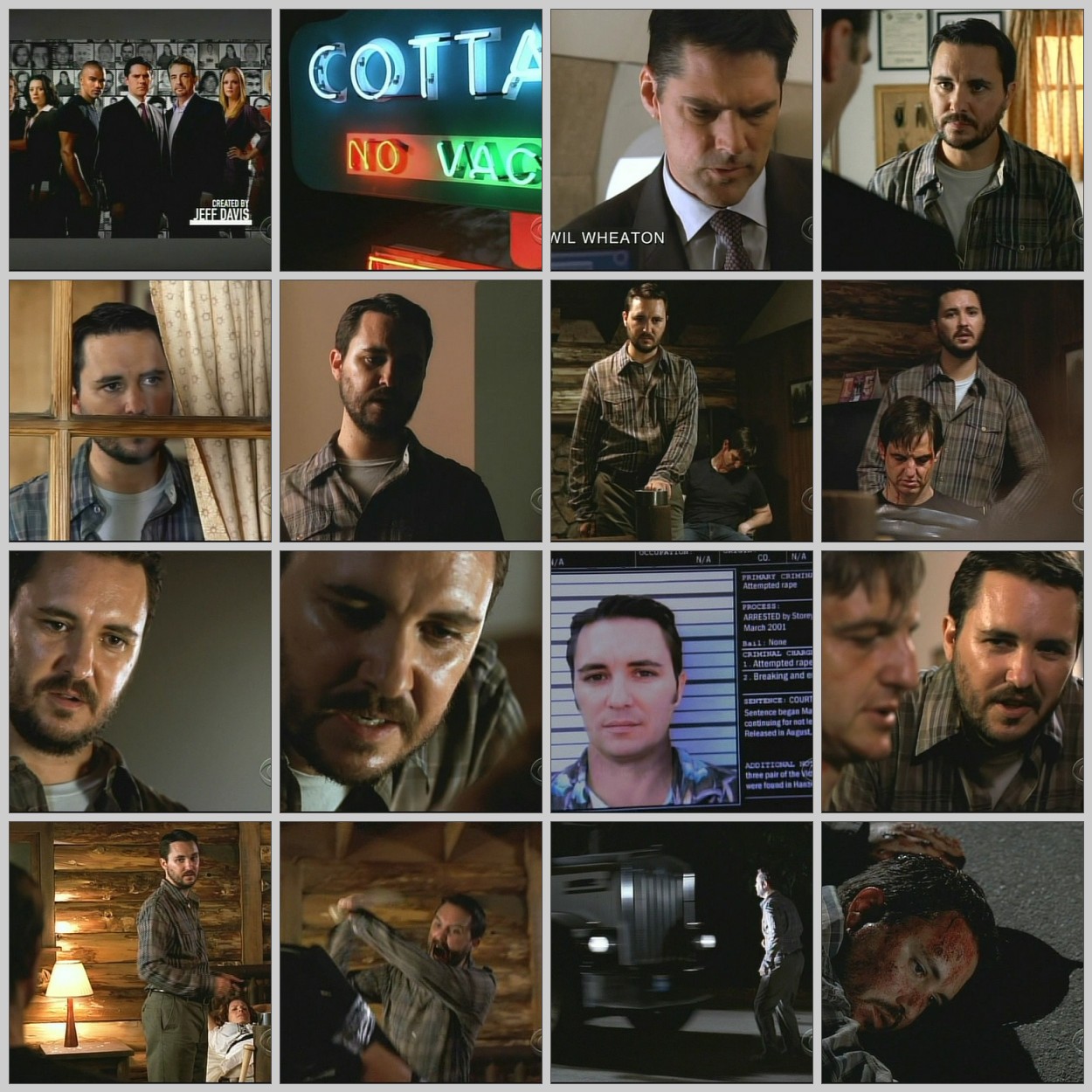The image is a collage composed of 16 distinct stills from the television series "Criminal Minds," created by Jeff Davis, featuring Wil Wheaton prominently. Organized in a 4x4 grid format, each small square encapsulates a different moment from the show. The top left square showcases the main cast standing together against a backdrop of mugshots, captioned with "Created by Jeff Davis." Adjacent to this is a close-up of a neon sign with partial text that presumably reads "No Vacancy." The majority of the squares predominantly feature Wil Wheaton, either alone or interacting with others. 

Wil Wheaton is depicted wearing a plaid shirt over a white T-shirt, and later in a suit. Scenes include him peering through a window, engaging in deep conversations in front of framed diplomas and golden curtains, and appearing younger in a mugshot. Dramatic moments portray him in a log cabin, interacting with someone tied to a chair, and ultimately, lying on the ground with a bloodied face. The detailed progression of images provides a glimpse into the intense narrative arc revolving around his character.